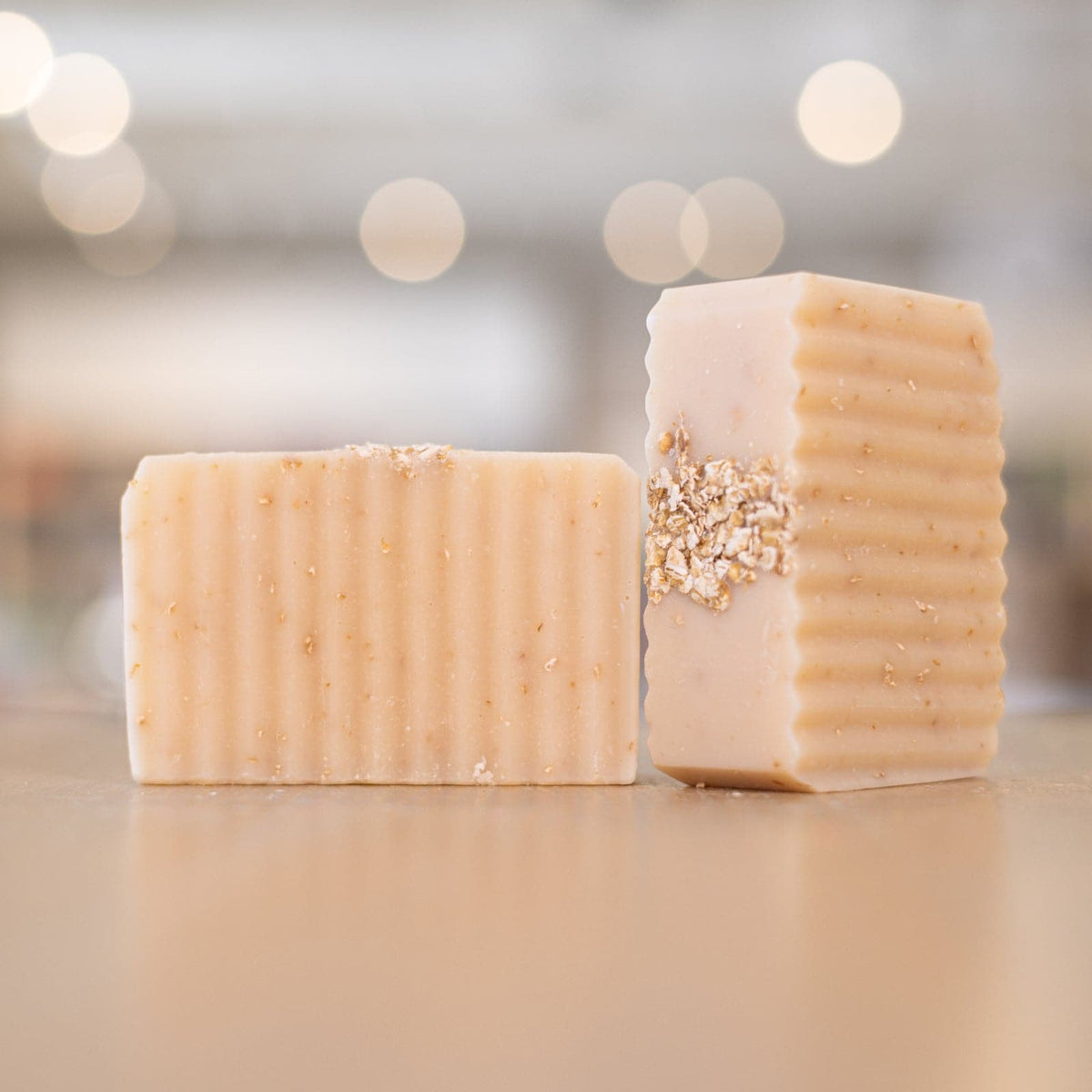This image features a beautifully styled promotional photo of two handmade soap bars displayed on a metallic pink table. The soap bars are a delicate peach color with a crinkle-cut texture along their edges. One bar is positioned vertically, showcasing the smooth top embellished with crunchy golden particles and what appear to be oats, likely for exfoliation. The other bar is oriented horizontally, allowing the side crinkle cut and the textured detailing within the soap to be visible. The creamy surface and blurred backdrop, adorned with soft white and peachy circles, enhance the airy, pastel aesthetic, highlighting the intricate design and artisanal quality of the soap.